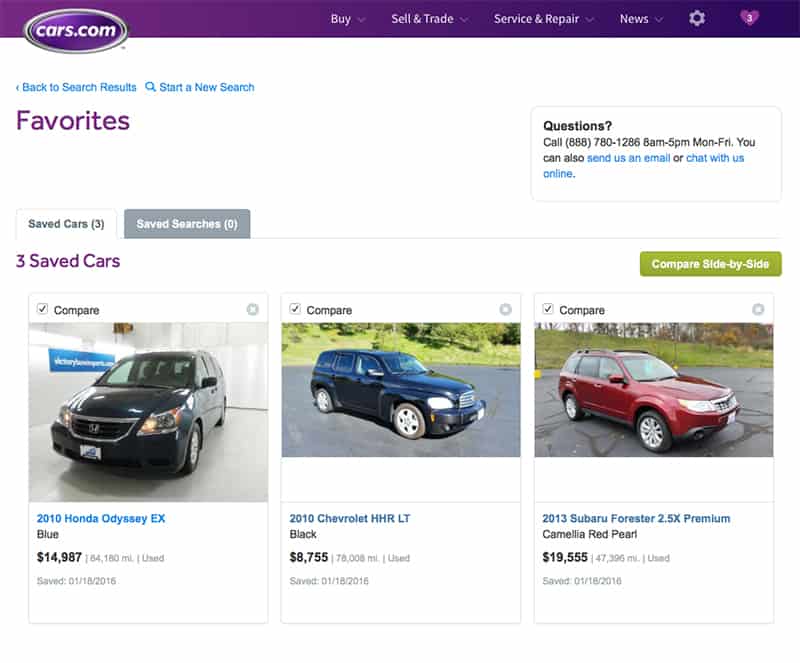Screenshot of a cars.com Website Favorites Page

In the upper left-hand corner of the screenshot, a purple oval featuring the "cars.com" logo is prominently displayed. The website's main navigation bar is visible at the top of the page with options listed from left to right: "Buy," "Sell & Trade," "Service & Repair," "News," followed by a cog icon for settings and a purple heart icon indicating the user's favorites, which is currently showing the number 3.

The user is currently on the "Favorites" tab, highlighted in purple in the upper left-hand corner. Located to the right of the tab is a contact information box that states, "Call 888-780-1286, 8 a.m. through 5 p.m. Monday through Friday." It also includes options to "send us an email" or "chat with us online."

The main section of the webpage displays three saved cars. From left to right, the details are as follows:

1. A 2010 Honda Odyssey EX in blue, priced at $14,987, with 64,160 miles. This car was saved on January 18, 2016.
2. A 2010 Chevrolet HHR-LT in black, priced at $8,755, with 78,008 miles. This car was also saved on January 18, 2016.
3. A 2013 Subaru Forester 2.5X Premium in Camellia Red Pearl, priced at $19,555, with 47,396 miles. This car was saved on January 18, 2016.

The layout of the webpage is clean and user-friendly, allowing easy access to the user’s favorite saved vehicles and contact information for further assistance.